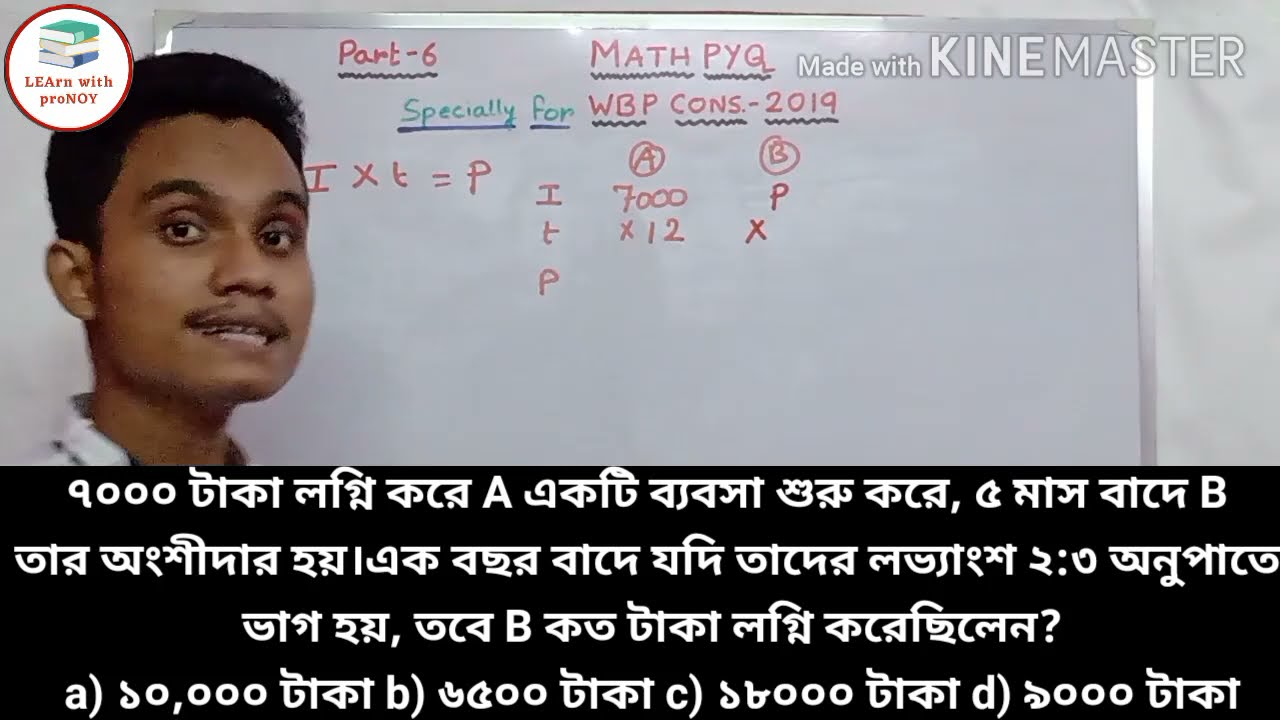This image appears to be a still from an educational video focused on math, specifically Part 6 of Math PYQ for WBCons 2019. The video seems to be hosted by a young man of East Indian descent, who appears to be in his late 20s. He has short dark hair and a thin mustache. The man is positioned on the left side of the image, and we can see him from the neck up as he speaks directly into the camera, smiling slightly.

Behind him is a large whiteboard with mathematical equations written in red and green marker. The top left corner of the image features a white circular logo with a red outline, containing an icon of three stacked books and the text "Learn with Pronoy." Additionally, the words "Made with KineMaster" are visible in the upper right corner.

The bottom third of the image is dominated by a large black text box filled with white text in an Indian script, including multiple-choice options labeled A, B, C, and D. This suggests the video includes practice test questions in a quiz or exam format. The background and the digital enhancements suggest that this image is a screen grab from a video optimized for online learning.